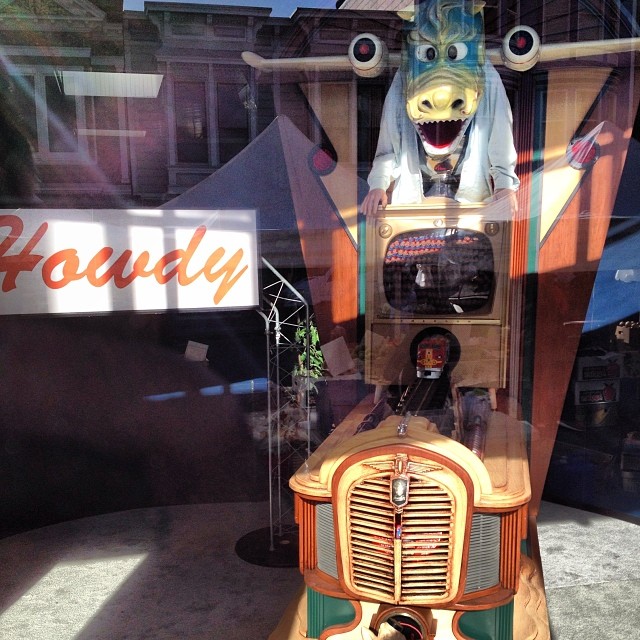The image showcases an eclectic display that resembles a whimsical tourist attraction or museum exhibit behind a window. Dominating the left side of the scene is a white sign with red, cursive text that cheerfully says "Howdy." The centerpiece of the display is an intriguing concoction of elements. At the base, there appears to be the front of a classic car, above which a train emerges dramatically from a hole in an old-fashioned TV set. Overseeing this surreal assembly is a figure with a human body clad in a white jacket. However, the figure's head is that of a blue and yellow dragon. To add to the fantasy, airplane wings seem to sprout either from the side of the dragon head or its back. The dragon-headed figure's hands grip the TV below, enhancing the bizarre and imaginative nature of the scene.